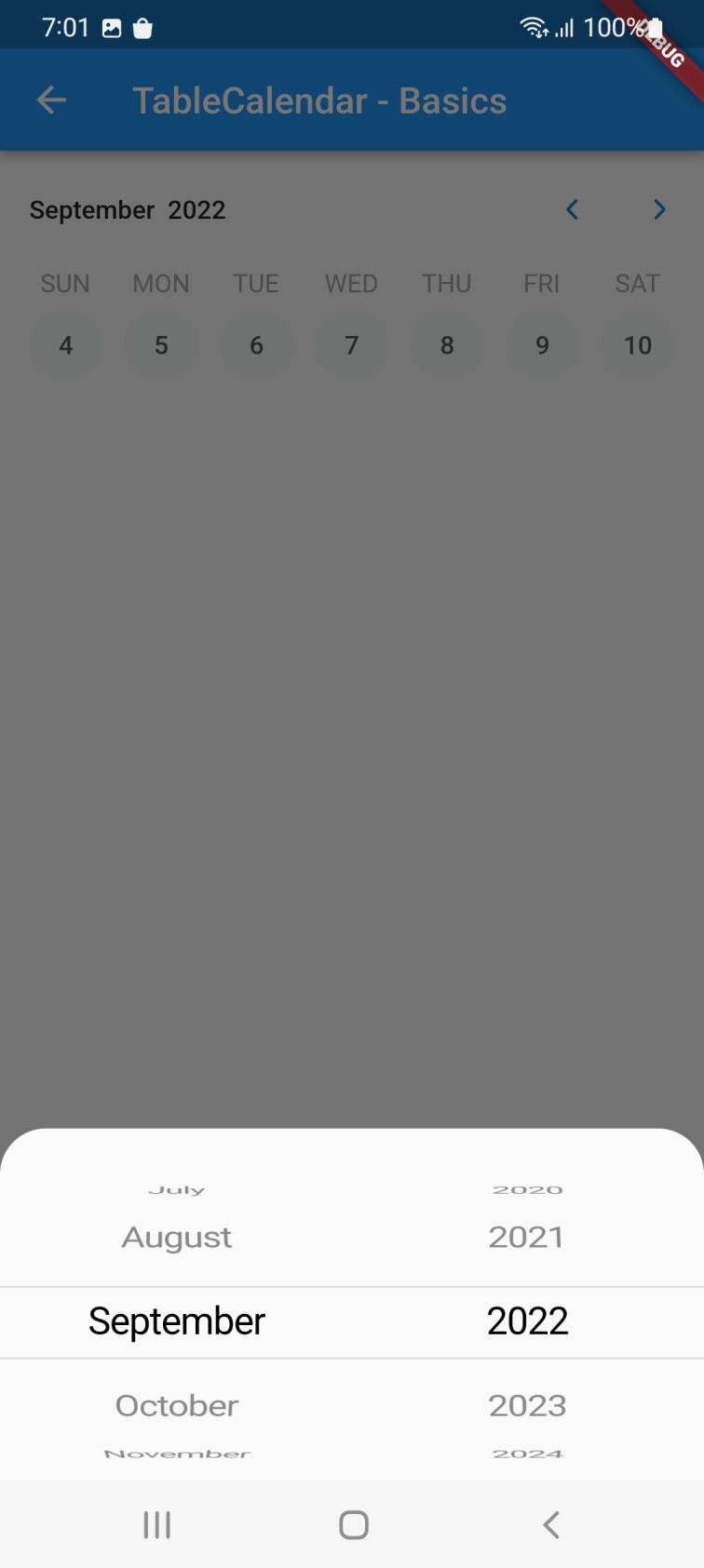This detailed caption describes the image of an iPhone screen displaying a calendar app:

The image showcases an iPhone screen that is fully charged at 100%, indicated at the top right corner. The time displayed is 7:01. Focused on the screen is a table calendar titled "Table Calendar Basics" written in blue, with a semi-transparent gray overlay providing additional information. The calendar month displayed is September 2022. Navigational arrows in blue allow the user to scroll left or right through the months. 

The calendar layout displays the days of the week from Sunday to Saturday, with the dates within the range starting on Sunday the 4th and ending on Saturday the 10th. Below this weekly layout, there is a gray space occupying the lower half of the screen.

In the upper section of the screen, there is additional navigation for months and years, listing July, August 2022, 2021, September, 2022, and October 2023 in black text with a scrollable view. The text "November 2024" appears faintly at the bottom, hinting at the continuation of the calendar.

Beneath the calendar, the familiar elements of an iPhone home screen interface are visible, including a home button and various icons. On the lower right, an arrow points left and there are three vertical lines, indicating menu options. A red banner stretches from one edge of the screen to the other in the upper-right corner.

This comprehensive view captures the intricacies and multi-layered navigation capabilities of the calendar app on an iPhone.